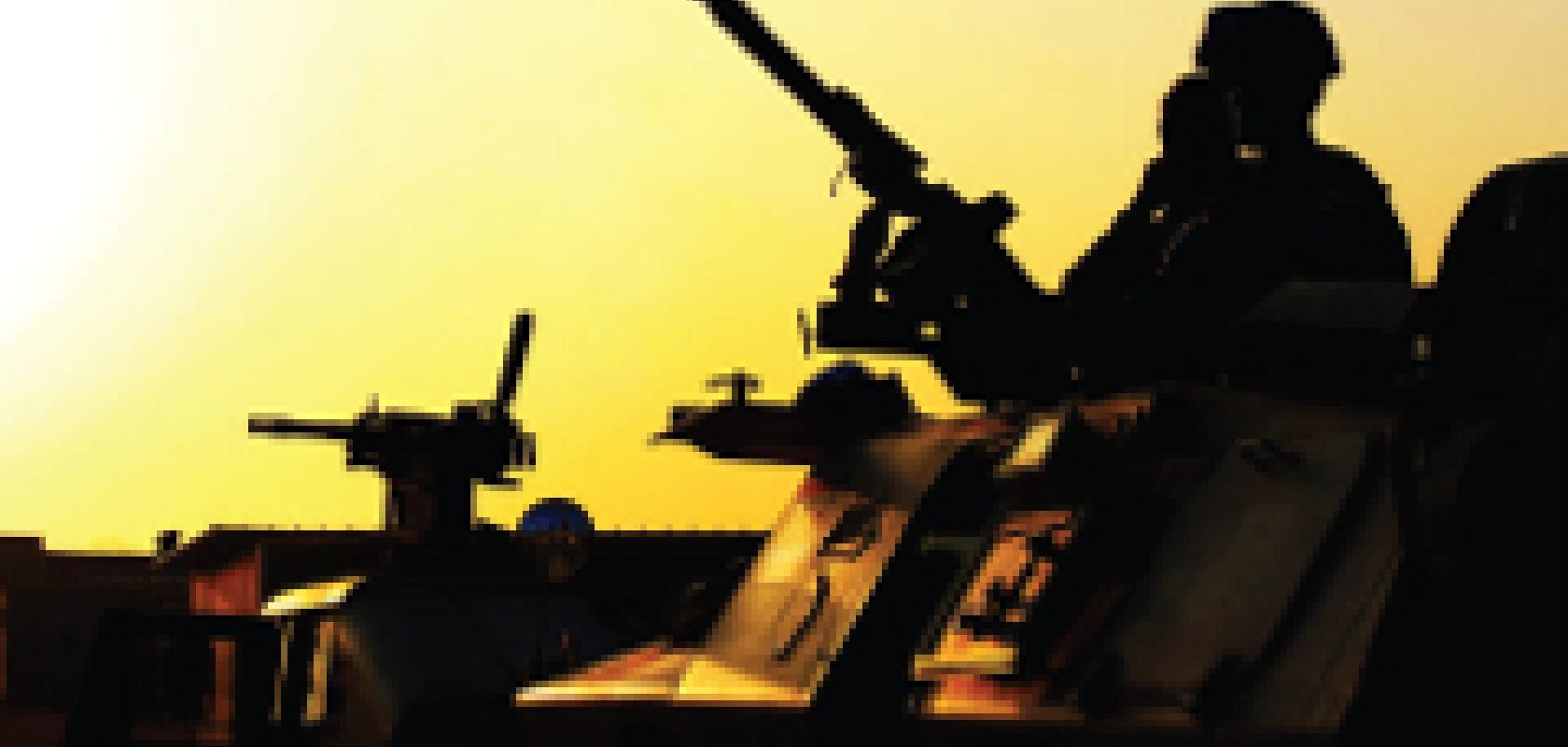The image is a heavily pixelated, low-resolution dusk shot depicting a military scene. At the center-right of the image, two soldiers, visible only as black silhouettes due to the low quality, are standing on top of a tan-colored tank. One soldier in the foreground seems to be manning a large machine gun mounted on the tank, which is angled upwards towards the sky. This soldier's face is obscured, possibly covered by a mask or helmet, adding to the silhouette effect. Next to him, towards the rear of the tank, a second soldier stands near another mounted weapon, though the lack of detail makes it difficult to discern his actions. The sky in the background is a dark yellow hue, with a bright white light from the setting sun visible in the upper left corner, casting a golden reflection on the tank. In the lower left corner of the image, another unmanned mounted weapon can be seen atop a dark structure, perhaps a roof or a building painted in red. The whole scene is against the backdrop of a silhouetted structure that might be a building or an industrial emplacement, contributing to the suggestion of a war zone or battlefield.